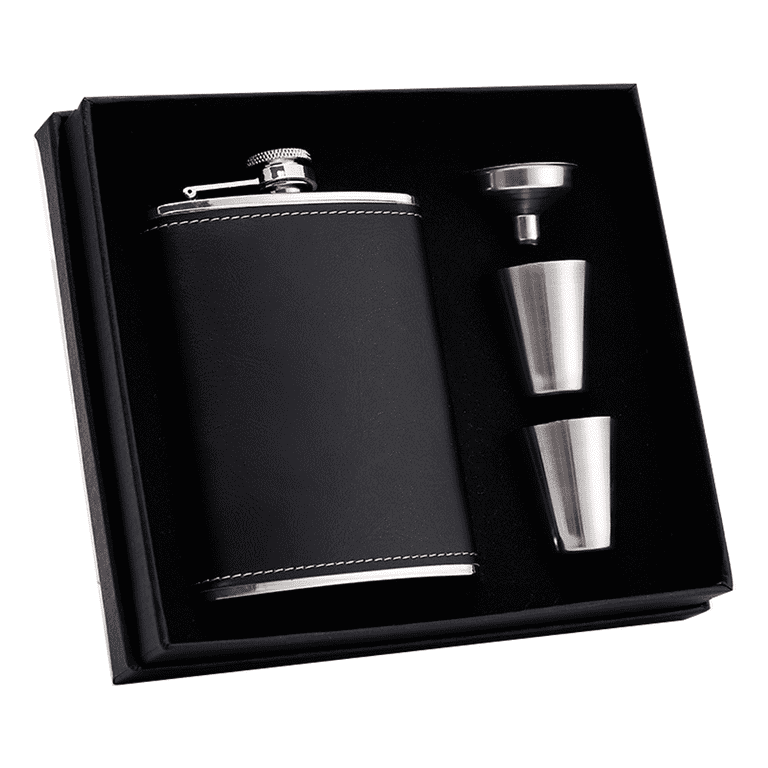This color photograph showcases an elegant gift set tailored for the sophisticated drinker. Nestled in a fitted black presentation box, the centerpiece is a striking, silver-looking flask adorned with a luxurious black leather cover, meticulously stitched in white. Complementing the flask are two gleaming silver shot glasses and an additional mysterious silver item that might serve as an alternative top for the flask. The entire ensemble is presented with the lid of the box positioned underneath, underscoring the set's readiness for gifting. The flask's placement on the left, alongside the three accompanying items, accentuates the visual appeal and functional design of this exquisite set. There are no visible writings, people, or animals in the image, allowing the focus to remain entirely on the sophisticated drinkware set.